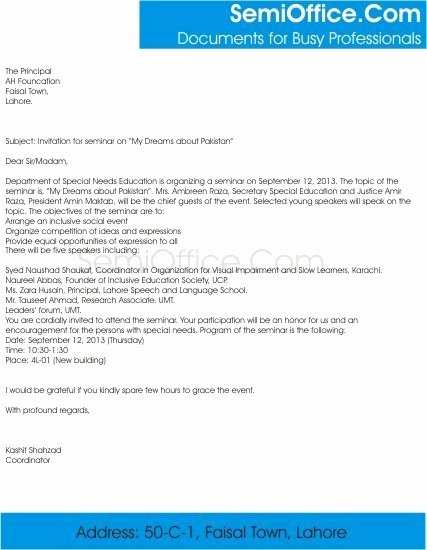The image depicts a formal letter, prominently featuring a header in the top right corner. The header contains a blue rectangle with the text "semioffice.com" and the tagline "Documents for busy professionals." The main body of the letter is printed in black font on a white page, with a visible grey watermark of "semioffice.com" across the document.

The letter is addressed to "The Principal, AH Foundation, Faisal Town, Lahore," with the subject line stating, "Invitation for Seminar on 'My Dreams About Pakistan.'" The letter is formal and begins with "Dear Sir/Madam," indicating a respectful and inclusive address.

The content details an upcoming seminar organized by the Department of Special Needs Education, scheduled for September 12, 2013. The seminar's theme is "My Dreams About Pakistan." The letter further mentions that Mrs. Avery Reza, Secretary, Special Education, and Justice Army Raza, President, Admin Madotab, will attend as the chief guests. 

It elaborates on the purpose of the seminar, highlighting objectives such as arranging an inclusive social event, organizing a competition of ideas and expressions, and providing equal opportunities of expression to all participants. The letter concludes by stating that there will be five selected young speakers presenting their views on the topic.

The document is meticulous in its presentation, aimed at inviting the principal to be a part of this significant educational and social event.